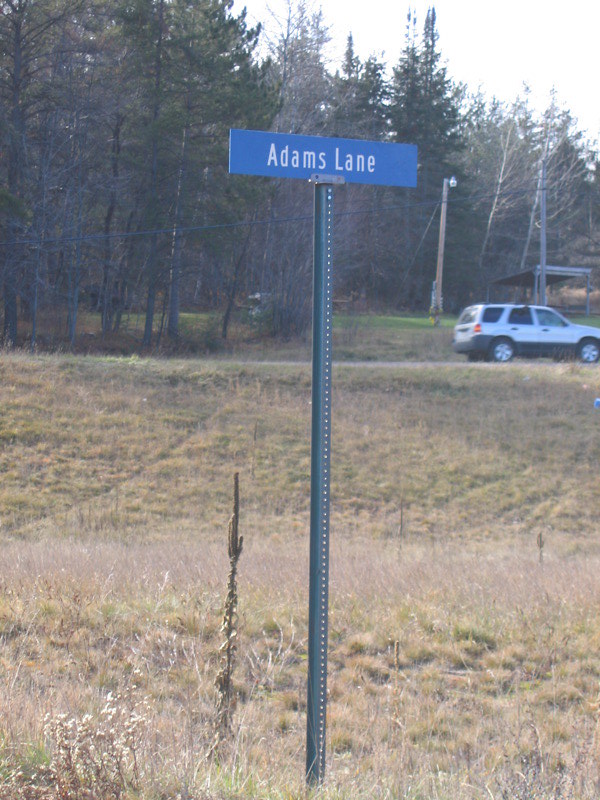This close-up image features a rectangular, blue road sign with white lettering that reads "Adams Lane." The sign is mounted on a metallic green pole with evenly spaced holes along its length, firmly planted in a grassy area. The foreground shows flat grass that gradually slopes upward to meet a road. On the road, a silver 4x4 sports utility vehicle is visible. Beyond the vehicle, more grass extends to the base of a mixture of tall trees. Some of these trees are evergreen, while others have lost their leaves, suggesting a seasonal transition. The focal point of the photograph is the Adams Lane sign on its distinct green post, set against the varied backdrop of roadside scenery.